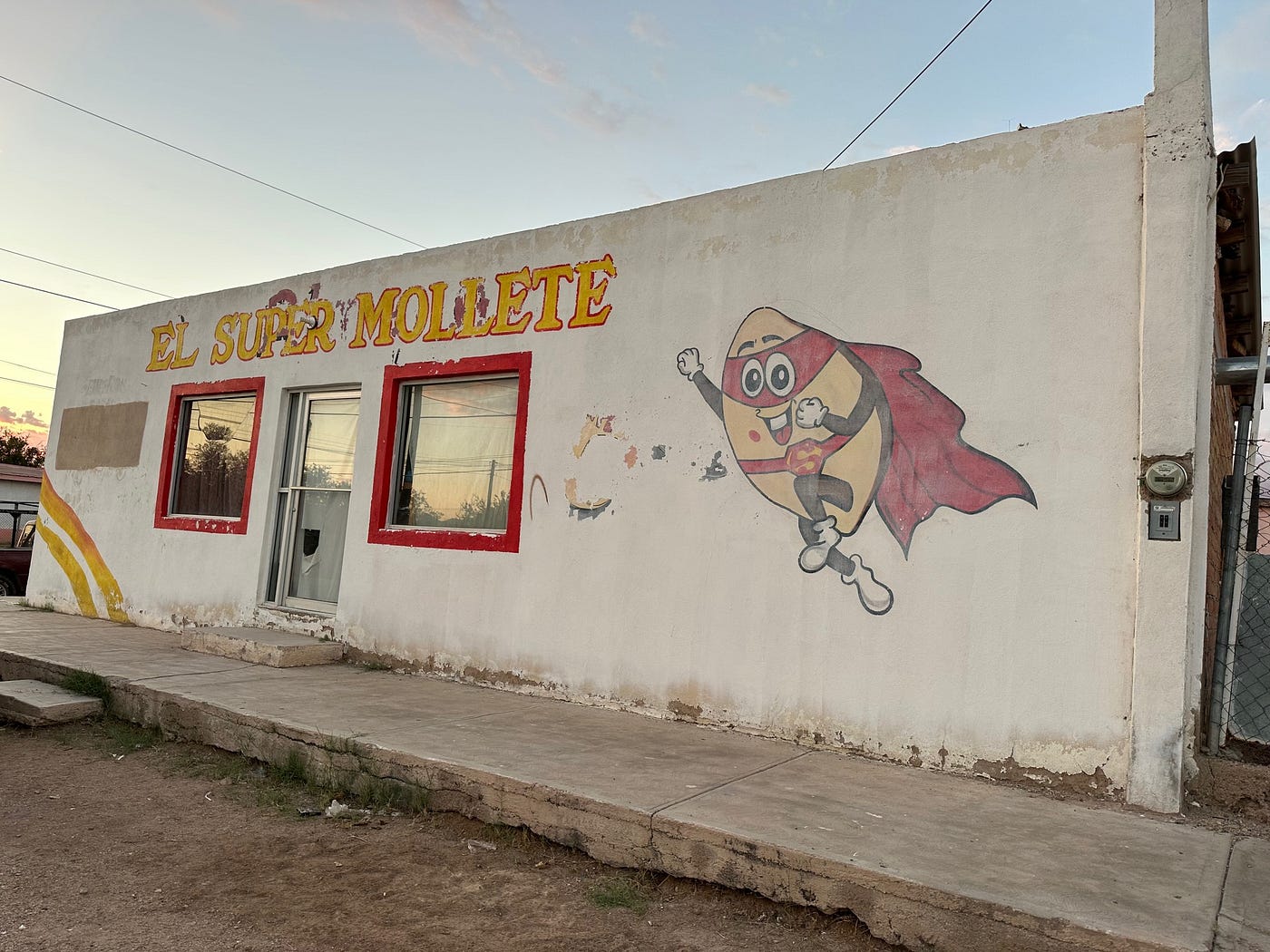This daytime photograph captures a worn, white concrete building with a slightly tapered structure. The facade features a central door flanked by two red-trimmed windows, all topped with the yellow-painted text "El Supermolet," M-O-L-L-E-T-E. The building’s exterior is dirty and aged, with notable disrepair. On the right side, a whimsical cartoon character is painted: a non-human figure resembling an avocado, complete with big googly eyes, a smiling mouth, a red mask around its eyes, a red cape, and a belt with an "S" emblem, depicted as if flying. To the left, two yellow stripes run down the bottom edge of the building. In front of the building is a crumbling sidewalk interspersed with patches of dirt, leading towards a chain-link fence at the far right. The sky shows shades of blue, suggesting the photo was taken as the sun was about to set.